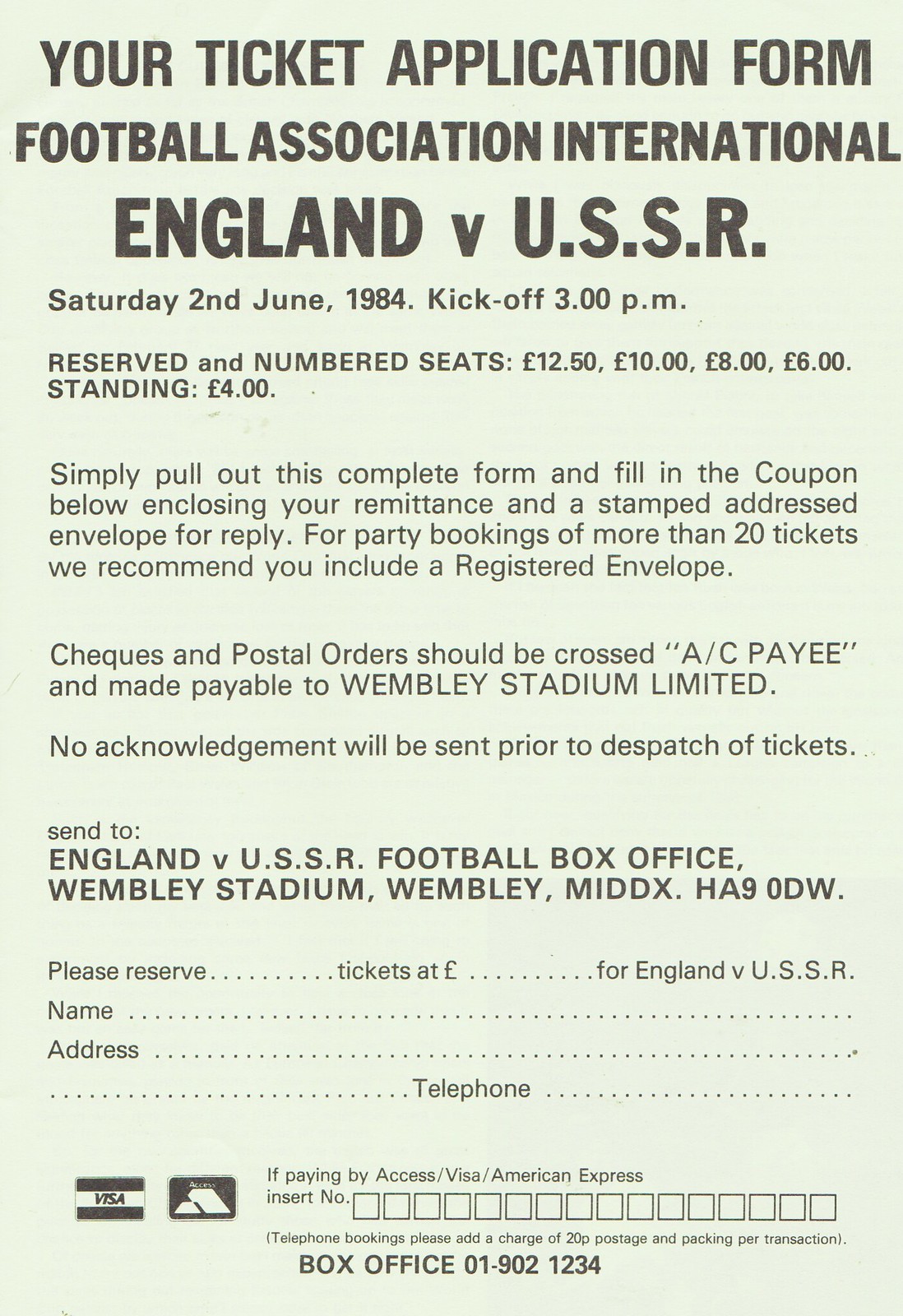This image features an older ticket application form for the Football Association International match between England and the USSR, scheduled on Saturday, 2nd June 1984, with a kickoff time of 3:00 PM. The background is a light blue or mint green color, adorned with bold black text. At the top, the largest text reads, "Your Ticket Application Form," followed by the match details: "Football Association International, England vs. USSR." Various ticket prices are listed: reserved and numbered seats at £12.50, £10, £8, £6, and standing tickets at £4.

The form includes detailed instructions: "Simply pull out this complete form and fill in the coupon below, enclosing your remittance and a stamped addressed envelope for reply. For party bookings of more than 20 tickets, we recommend you include a registered envelope. Checks and postal orders should be crossed ACP and made payable to Wembley Stadium Ltd. No acknowledgment will be sent prior to dispatch of tickets."

At the bottom, there is a section to fill in details for reserved tickets, including a line that reads, "Please reserve ____ tickets at £____ for England vs. USSR," as well as fields for name, address, and telephone number. Symbols for Visa and other payment methods are present. If paying by Access/Visa cards, you need to include your card number. Telephone bookings incur a 20p charge per transaction for postage and packaging, and the address for submission is listed as "England vs USSR, Football Box Office, Wembley Stadium, Wembley, MIDDX, HA9 0DW."